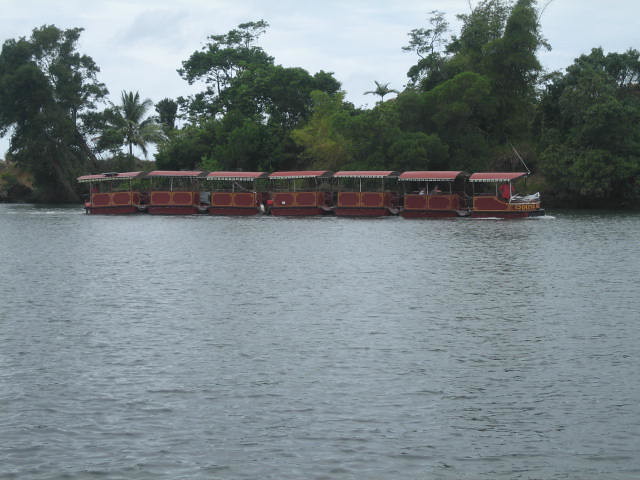This color photograph captures a serene water scene, featuring a train-like water vehicle on a river with small ripples on the dark blue surface. In the foreground, the water spans up to just beyond the middle of the image. The vehicle, which resembles a series of connected huts or water taxis, consists of seven parts. Each part is adorned with red roofs and red paneling with yellow lines in between, adding a striking contrast against the grey-blue sky. The leading section, which is slightly longer and houses the pilot, sports some Asian writing in gold. The vehicle appears to be ferrying people, possibly on a sightseeing tour. The backdrop is completed with tall, lush green trees, including both regular and pine varieties, under an overcast sky.